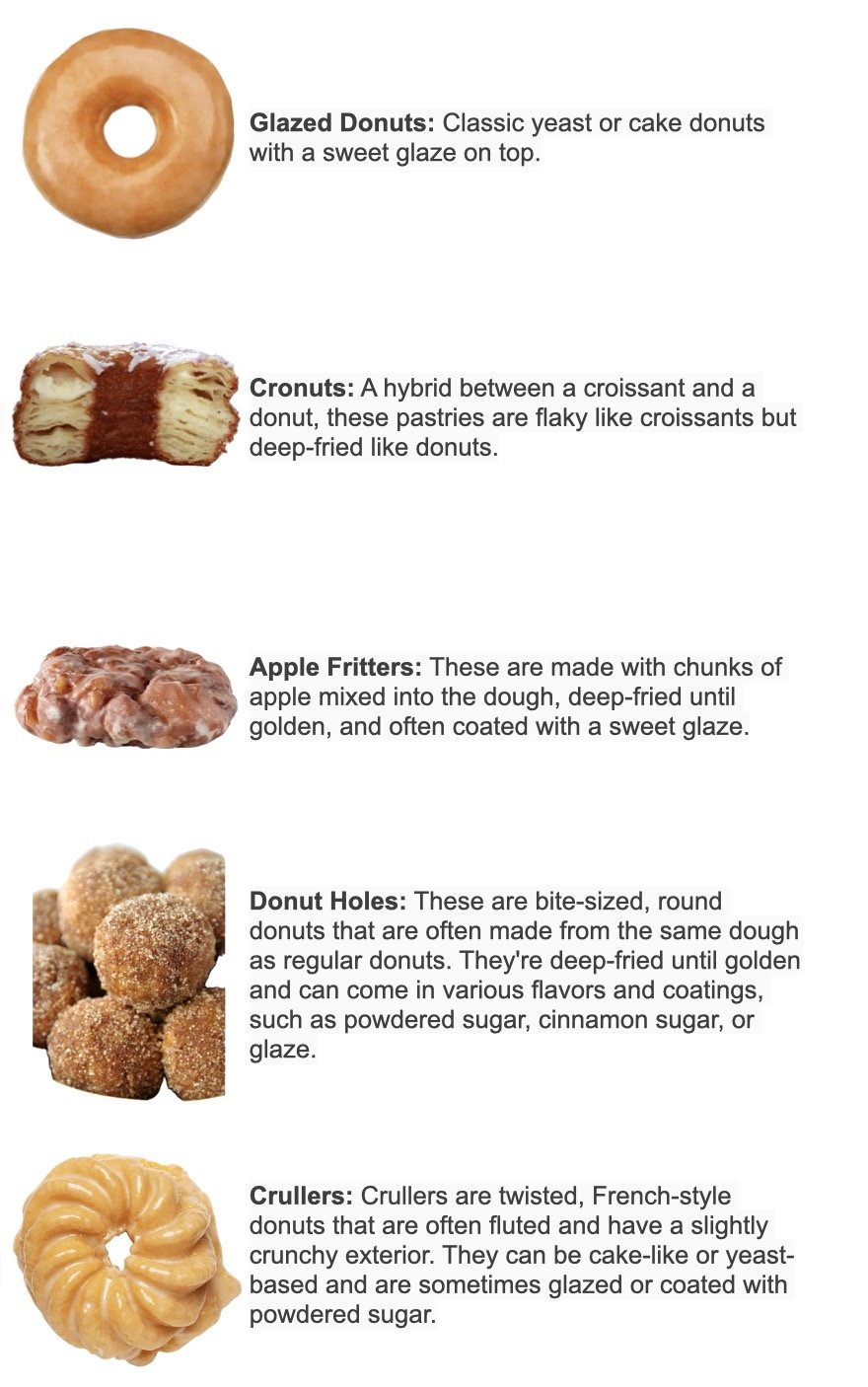This illustration depicts a variety of five different doughnut products against a white background. At the top is a classic glazed doughnut, a golden-brown treat with a sweet glaze that can come as either yeast or cake-based. Below that is a cronut, a hybrid of a croissant and a doughnut, showcasing a flaky, layered interior with a deep-fried, golden exterior. Next is an apple fritter, characterized by its irregular, lumpy shape with visible chunks of apple, deep-fried to a rich golden brown and often glazed. Further down are doughnut holes, small, round bites made from regular doughnut dough, deep-fried until golden and available in various coatings like powdered sugar, cinnamon sugar, or a simple glaze. At the very bottom are crullers, twisted French-style doughnuts known for their fluted appearance and slightly crunchy exterior, which can be cake-like or yeast-based and sometimes finished with a glaze or powdered sugar.